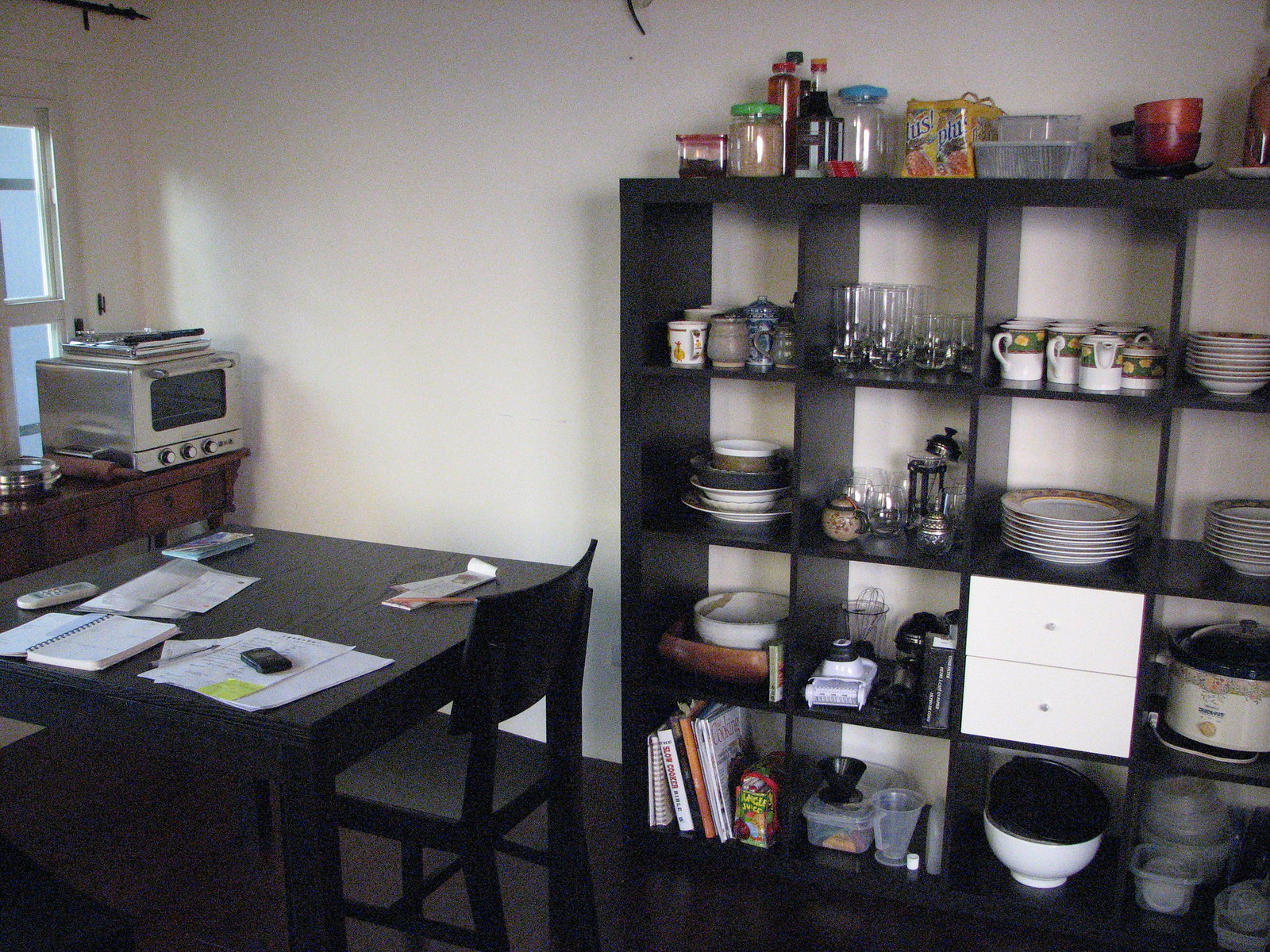The photograph captures a combined living and kitchen area, focused on a blank white wall. On the left side of the image, there's a window frame just before the corner, beneath which sits a small wooden desk. Atop this desk is an aluminum pie warmer, accompanied by a wooden rolling pin. Further left, a black table with a wood grain pattern stands, a wooden chair tucked neatly under it on the right side. Scattered across the table are various papers and documents, along with a small black mobile phone resting atop one of the paper stacks. 

Against the white wall, a black cube-style shelf with four rows of four square spaces is prominently featured. The top of the shelf is cluttered with numerous containers and bottles. Each cube space holds a variety of kitchen items, including plates, cups, and ceramics. In the bottom left corner cube, books are stacked, while the third cube from the left on the third row contains two white drawers.